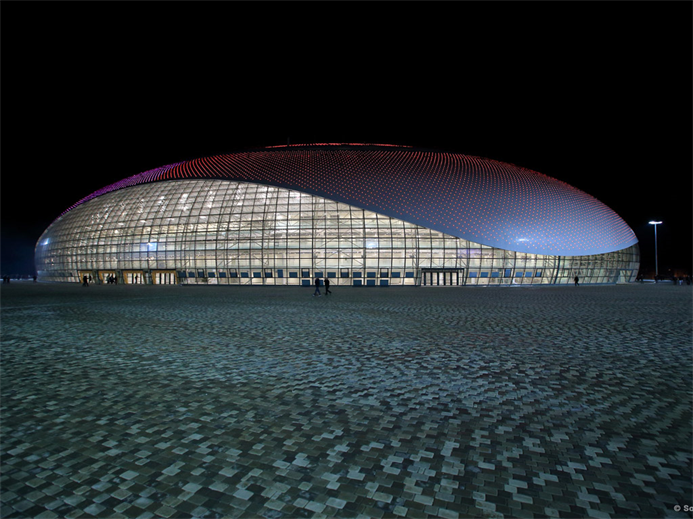The nighttime photo captures the Bashoy Ice Dome in Russia, an architecturally striking sports stadium with an innovative and modern design. The dome has an overall egg-like, rounded shape, reminiscent of a water droplet sitting on the ground. The front facade features a grid of clear windows, while the top is a gray surface that curves downward, blending seamlessly with the structure. At night, the exterior is illuminated by neon red and purple lights, creating a dotted pattern across the blue surface. The image is taken from a distance, approximately 100 meters away, showcasing the arena's full grandeur. The foreground consists of multi-colored pavers arranged in a tiled pattern. The sky is completely black, providing a stark contrast to the brightly lit dome, and a street lamp can be seen glowing in the distance. A few people are visible walking in front of the arena, adding a sense of scale to the scene.